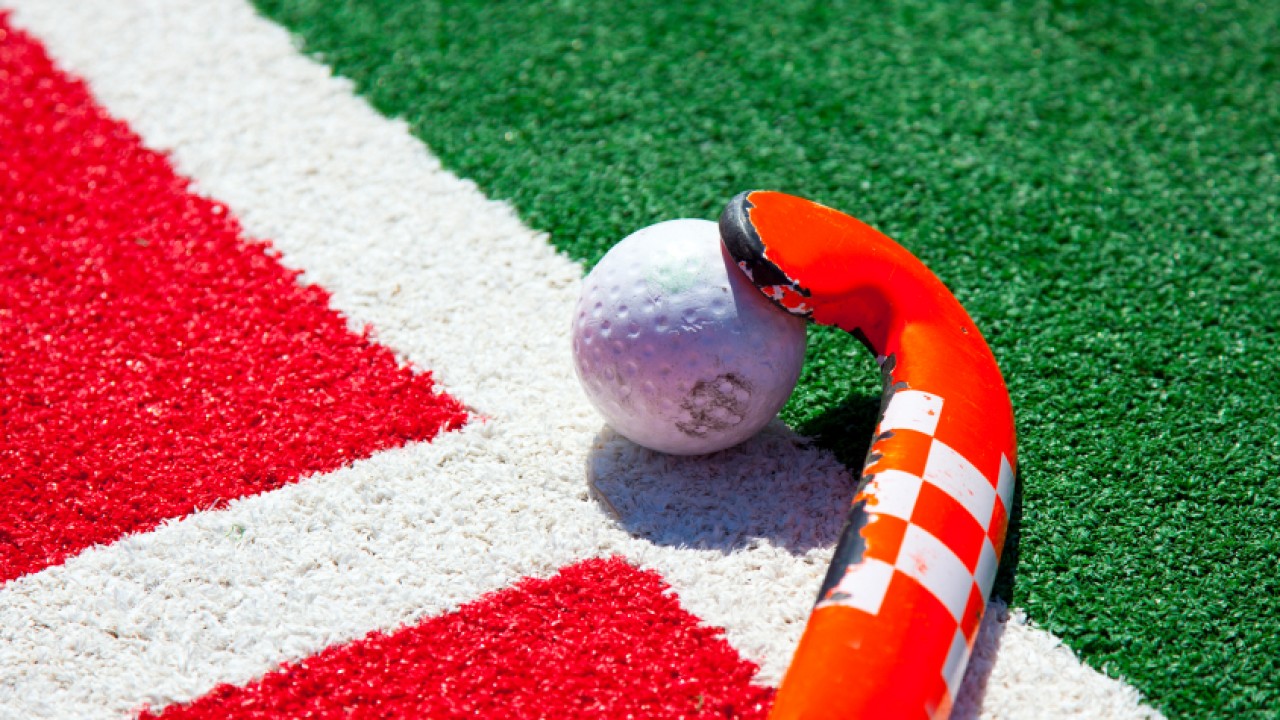In this close-up, color outdoor photograph, we see a well-worn, orangish-red field hockey stick with a white checker pattern at its base, positioned on an artificial turf field. The field features a distinctive pattern with a diagonal white line running from the lower right to the upper left corner, creating sections of different colors: red in the lower left, green in the upper right, and white intersecting in a T-shape near the center. Resting against the brightly colored and curved "J" shape of the stick is a used white field hockey ball. Sunlight casts a shadow of the ball, emphasizing its texture and the field's patterns. The extensive use visible on both the ball and the stick highlights their active role in the game.